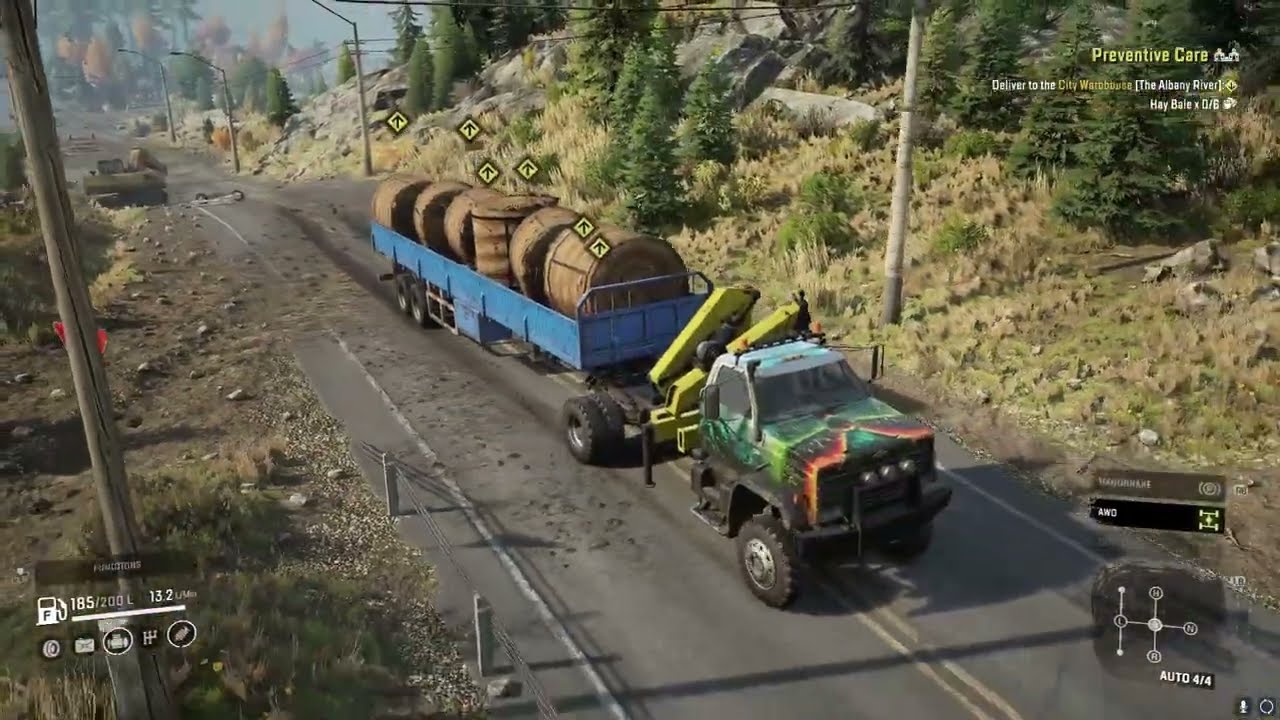This screenshot from a truck driving simulation video game features a large truck with a tie-dye and flaming green paint job hauling a blue trailer filled with massive brown bales of hay. The truck is unusually positioned in the center of a two-lane road with a yellow double divider, likely indicating something has gone wrong. The road is flanked by a rugged, wooded landscape with a hill and scattered trees on the right and dirt patches with pebbles on the left. This daytime scene is rendered with details such as lampposts lining the road and debris scattered across the asphalt. The user interface includes various on-screen overlays: a "preventive care" message and other game instructions at the top right, a transmission schematic at the bottom right, and fuel and speed indicators at the bottom left, enhancing the immersive experience of hauling through a mountainous terrain.